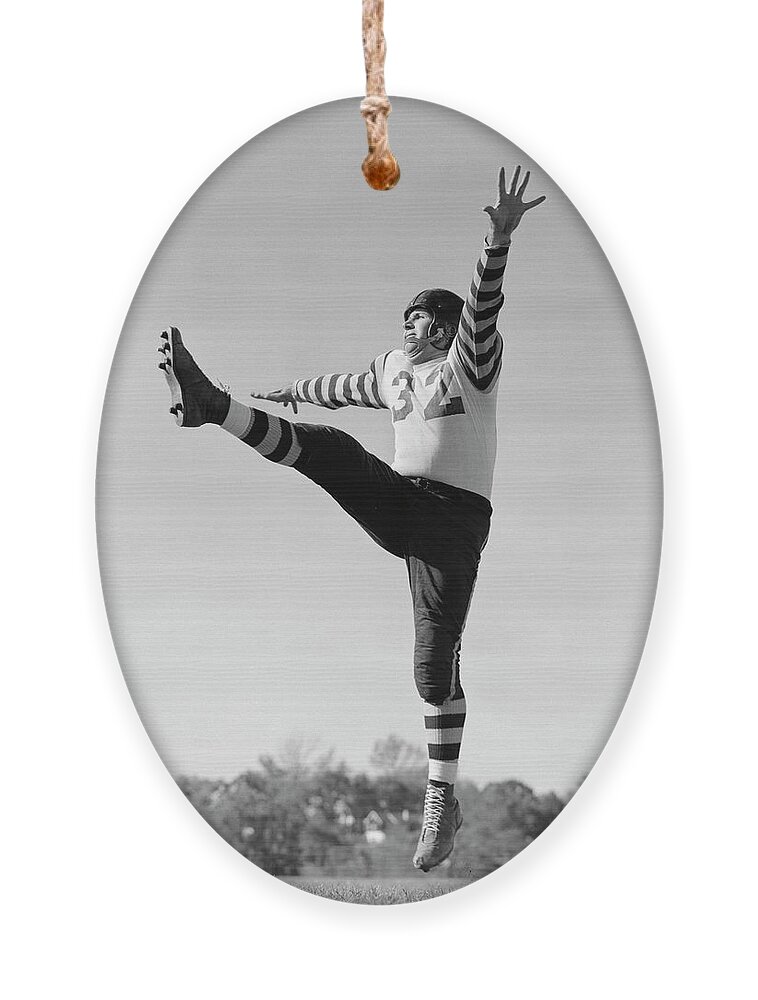This is a black-and-white image superimposed on an oval-shaped item, possibly porcelain or wood, and adorned with a hanging string at the top, likely designed to serve as an ornament, possibly a Christmas ornament. The image features a vintage football player, wearing a leather helmet and a striped jersey with the number 32 prominently displayed. The player is captured mid-action, with his right leg extended as if he has just kicked a football, both arms outstretched in a T-pose. He is elevated off the ground, and wears old-fashioned cleats. In the background, the scene includes grass and distant trees, adding to the historical ambiance of the photograph.